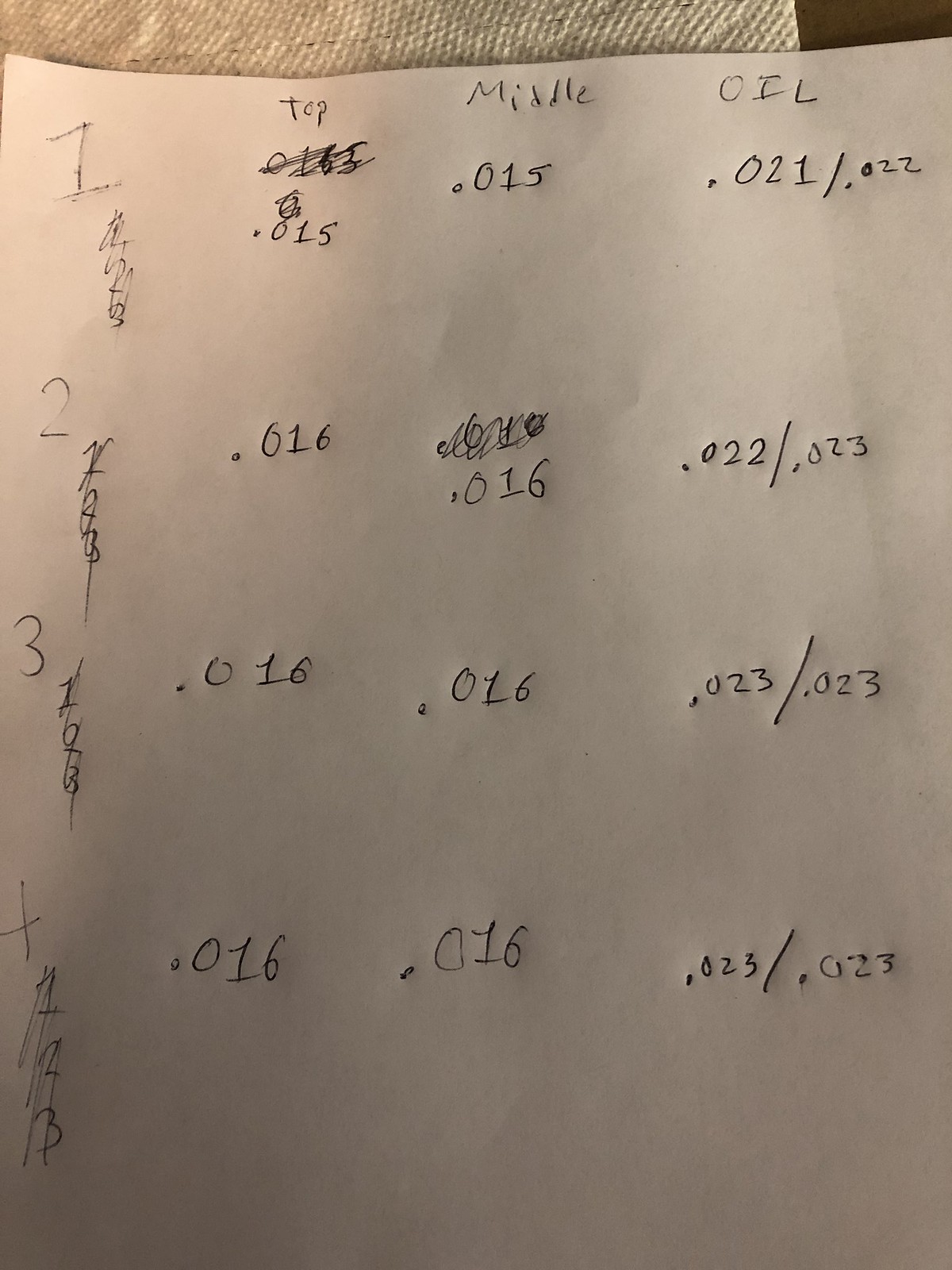This image features a white piece of paper displaying various sets of numbers and letters. The paper casts a subtle shadow towards the bottom and middle, indicating that the shadow might be from the person taking the photo. The paper sits atop a very dark tan surface, but the background is visible only at the top edge and in the top right-hand corner, where it appears dark.

On the left side of the paper, numbers are listed vertically from 1 to 4. At the top of the paper, headers divide the content into three sections labeled "Top," "Middle," and "Oil." Each section contains rows of numbers:

- Under "Top," the numbers are as follows:
  - 0.015
  - 0.016
  - 0.016
  - 0.016

- Under "Middle," the numbers repeat similarly:
  - 0.015
  - 0.016
  - 0.016
  - 0.016

- Under "Oil," the rows contain pairs of numbers separated by slashes:
  - 0.021 / 0.022
  - 0.022 / 0.023
  - 0.023 / 0.023
  - 0.023 / 0.023